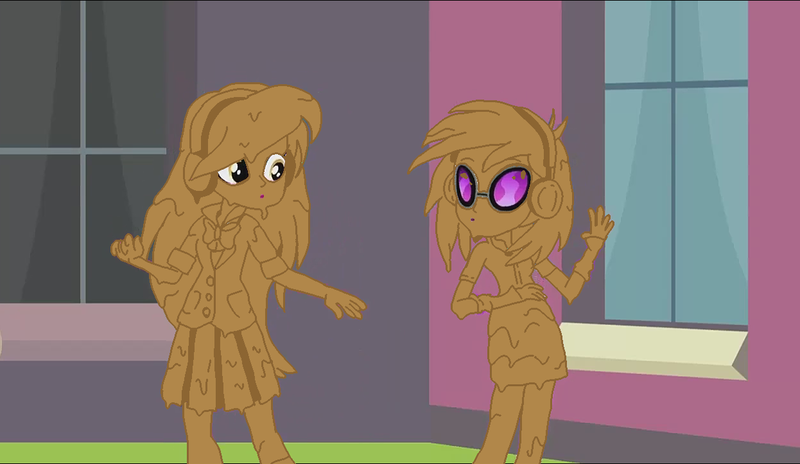In this cartoon drawing, two female characters are depicted, covered in a uniform, brownish-orange goopy fluid that envelops their entire silhouette. The character on the right is adorned with bright purple goggles featuring a distinctive pink wave and dark black edges, lending a striking contrast to her brown-toned figure. She wears a short dress and pants, and has long hair. To her left, another woman, also covered in the same brownish-orange fluid, has large, white eyes with yellow stripes. She is dressed in a shirt, skirt, and bow tie, and her long hair flows down her back. Both characters have headphones similarly coated in the fluid. They stand on a green floor, within a room that sports different colored walls: a gray wall behind the woman on the left and a pink wall behind the woman on the right. Each wall features a window; the left window has a light purple sill, while the right one has a white sill. The two women appear to be interacting with each other, likely engaged in conversation or a shared activity, with hands raised in expressive gestures.